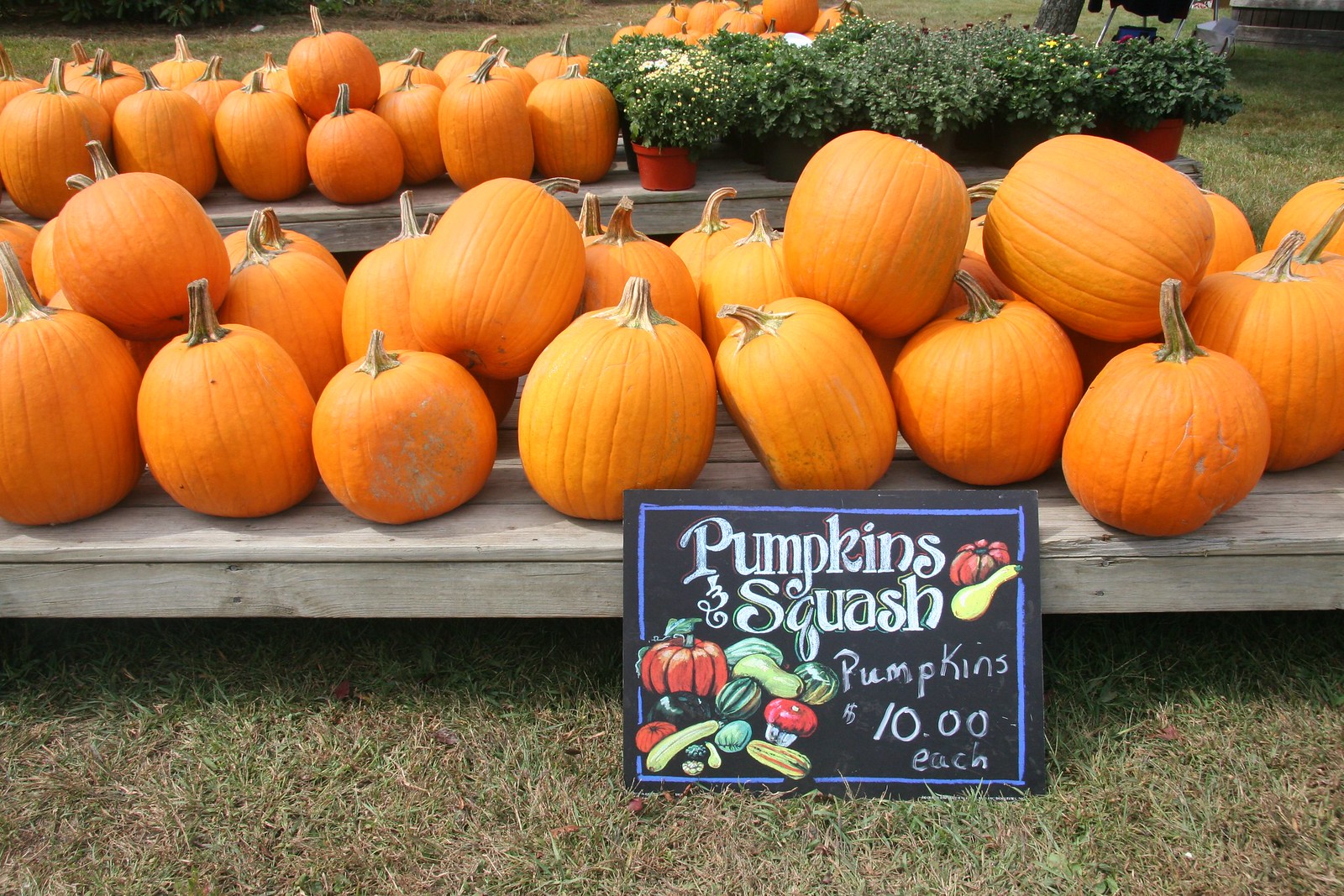The photograph depicts an outdoor setting featuring an array of bright orange pumpkins displayed on long, gray wooden benches. The benches are slightly elevated, about a foot off the ground. The nearest bench is entirely covered with pumpkins of varying shapes and sizes, some round and some oblong, many arranged upright with their stems pointing up. Leaning against this bench is a black chalkboard sign bordered with a purplish-blue line. The sign reads in large white text, "Pumpkins and Squash, Pumpkins $10 each," and is adorned with colorful illustrations of various produce, including pumpkins, squash, watermelons, tomatoes, and mushrooms. The bottom quarter of the image shows a stretch of green and brown grassy ground. 

In the background, another gray wooden bench is visible, with more pumpkins stacked on its left side and several pots of plants on its right side. These plants feature white, purple, and yellow flowers. The scene extends into more green grass and additional pumpkins stacked towards the top edge of the image.